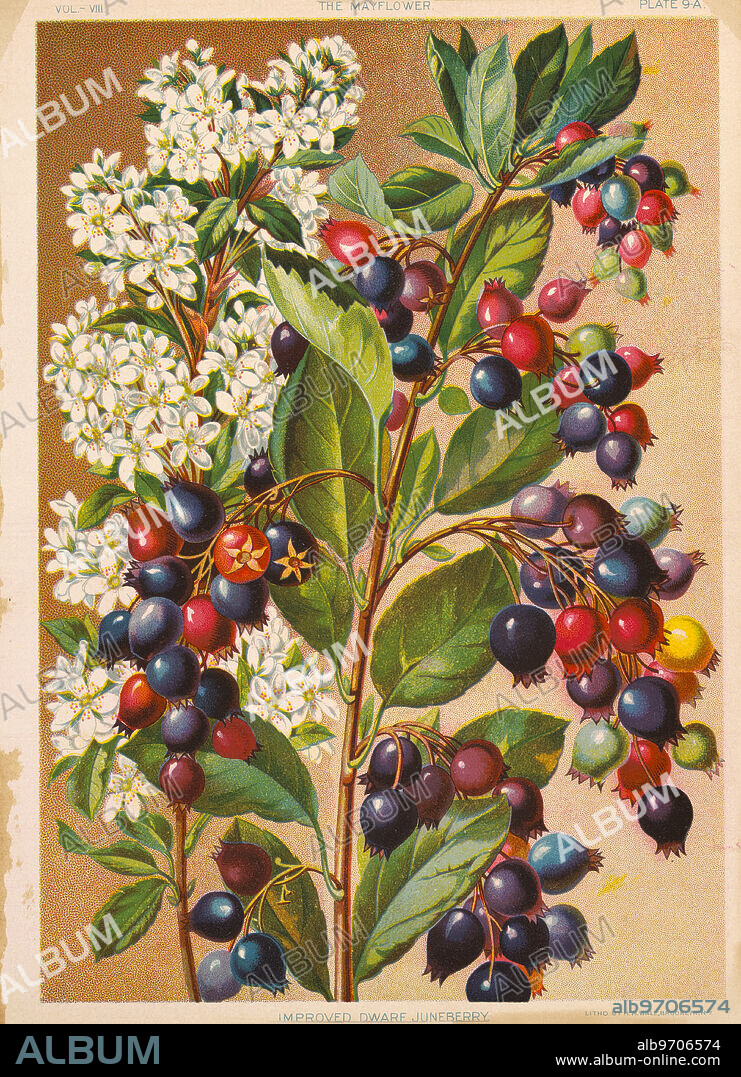The image depicts an oldish painting, possibly from the 1940s or 1950s, of a plant laden with berries and small white flowers. The plant's berries vary in color from red, dark blue, light blue, purple, yellow, green, to off white, suggesting different stages of ripeness or the artist's use of creative license. The plant features brown twigs with green leaves, and the white flowers are prominent on one of the stems. The painting has a brown background and a tan border with a black bottom edge. Watermarks reading "album" are scattered across the image, and the bottom right corner is stamped with "ALB 970 6574" alongside the URL www.albumonline.com. This painting is rendered in a delicate and washed-out style, reminiscent of vintage postcards.